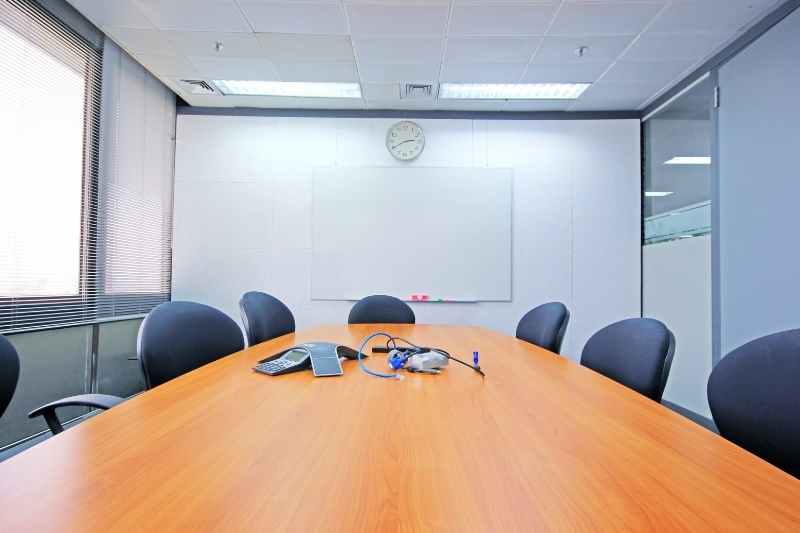This photograph depicts an empty business meeting room illuminated by ceiling lights. The room features a long, brown wooden table surrounded by seven dark green chairs. The table is neatly arranged with conference call equipment, including wires, buttons, and a calculator. On the front wall, which is white, there is a clock displaying 2:35 positioned above a dry erase board. The board is outfitted with red and green markers. On the left wall, the windows, adorned with blinds, allow daylight to stream into the room, enhancing its bright and professional atmosphere.